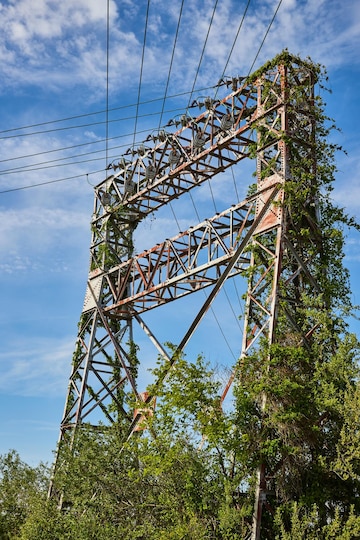The image depicts an aged and rusted electrical tower, resembling the lower section of the Eiffel Tower with crisscrossing metal reinforcements similar to bridge supports. This structure is heavily overgrown with vegetation, including bushes, vines, and trees, which are winding their way through its metal framework. There are approximately 6 to 12 power cables extending from the tower in various directions, with some appearing to crisscross near the top. The scene is set against a bright blue sky with scattered gray and white clouds, suggesting a clear morning or afternoon. Despite the evident wear and extensive rust, the wires indicate that the tower may still be in use, although it is clearly in need of maintenance. The abundance of greenery enveloping the base and ascending through the structure emphasizes its long-standing neglect.